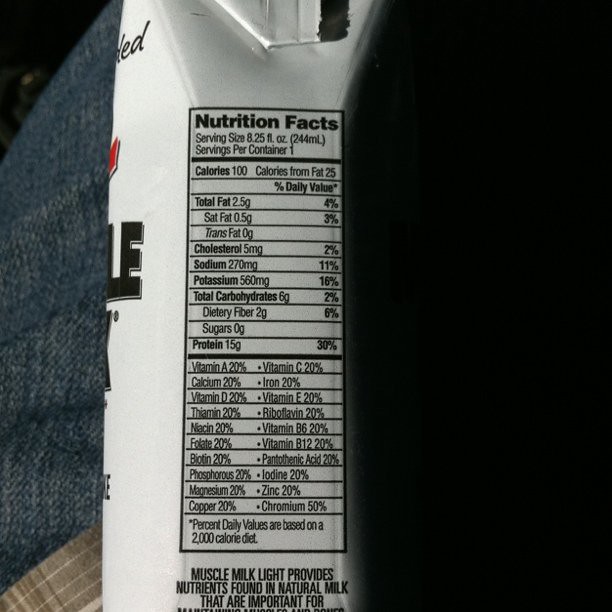The photograph is a close-up of the side labeling of a Muscle Milk Light juice box. The white rectangular container, positioned on someone's lap, shows detailed nutrition facts. On the left edge of the image, part of the person's jeans and a tan plaid shirt are visible. The right side fades into a shadowy void. The nutrition facts indicate the product has 100 calories, 2.5 grams of total fat, 0.5 grams of saturated fat, 0 grams of trans fat, 5 milligrams of cholesterol, 270 milligrams of sodium, 560 milligrams of potassium, 6 grams of total carbohydrates, 2 grams of dietary fiber, 0 grams of sugar, and 15 grams of protein. Below these, a comprehensive list of vitamins and minerals shows most at 20% daily value, except chromium at 50%. The bottom text partially reads, "muscle milk light provides nutrients found in natural milk that are important for," but the rest is cut off.